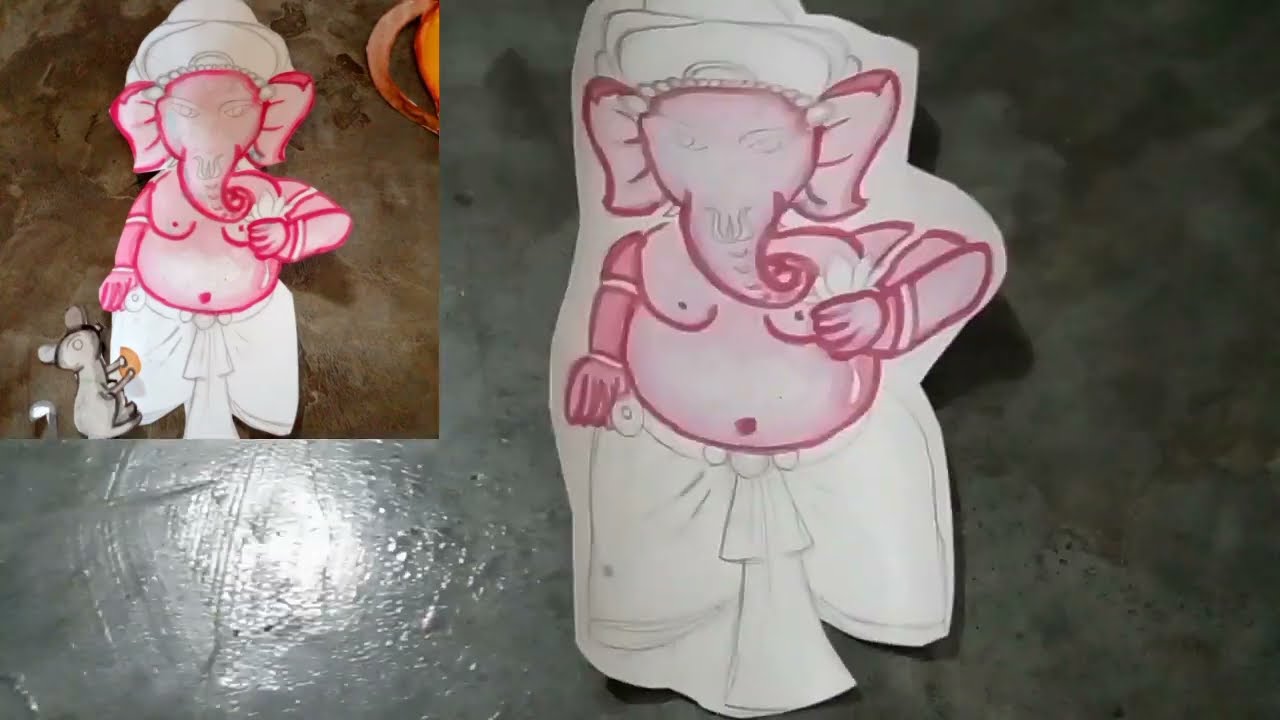The image features a detailed drawing of a pink elephant depicted twice – once in the main section and once in the upper left corner. The primary depiction of the elephant is centered on a shiny, dark gray background that reflects light in the bottom left corner. This pink elephant is adorned with a white headpiece, potentially a turban or headdress, decorated with pearl-like beads between its ears. The elephant's eyes are gray, and detailed gray writing extends from above its nose down its trunk, which gracefully twirls to the right. Human-like arms are part of the elephant's anatomy, each adorned with two white bands — one on the upper shoulder and one at the wrist. The right arm is held up over its chest, displaying a white flower. The elephant is shirtless, showcasing white strings around its arms below the shoulders, a large belly with a dot representing a belly button, and white, flowy pants or a skirt cinched by a belt with a white circular buckle.

In the upper left corner, the same elephant is depicted on a brown background, this version showing a deeper, more vibrant pink. Another notable difference in this segment is the presence of a gray mouse at the bottom, pressing its feet against the elephant's dress, near a brown spot. Additionally, this smaller depiction features the planet Saturn with its rings encircling it in the uppermost corner.